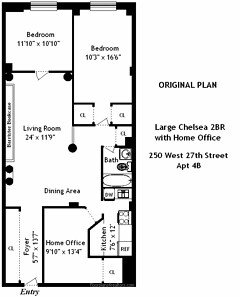[Original Floor Plan] "Large Chelsea Two-Bedroom with Home Office"

The floor plan of this house is presented on a black and white background, labeled "Original Plan, Large Chelsea Two-Bedroom with Home Office." The entrance opens into a foyer that seamlessly connects to the dining area. Directly to the right of the foyer, you'll find a functional kitchen. Moving straight ahead from the foyer, you enter a spacious living room, perfect for family gatherings.

Toward the front of the house, the layout becomes more compact with the home office, utility room, and bathroom clustered together, efficiently utilizing the available space. The rear of the house features two cozy bedrooms. The larger of the two measures 10 by 16 feet, while the smaller one is 11 by 10 feet. Notably, the smaller bedroom appears to lack a closet, indicating limited storage options throughout the house. 

The floor plan does not show a clear back door; there is a possible exit off the kitchen, suggesting that the house may have only one main entry point, which could be a concern for some potential homeowners.

Overall, this detailed layout provides a clear picture of the house’s structure, highlighting its strengths and potential areas for improvement.